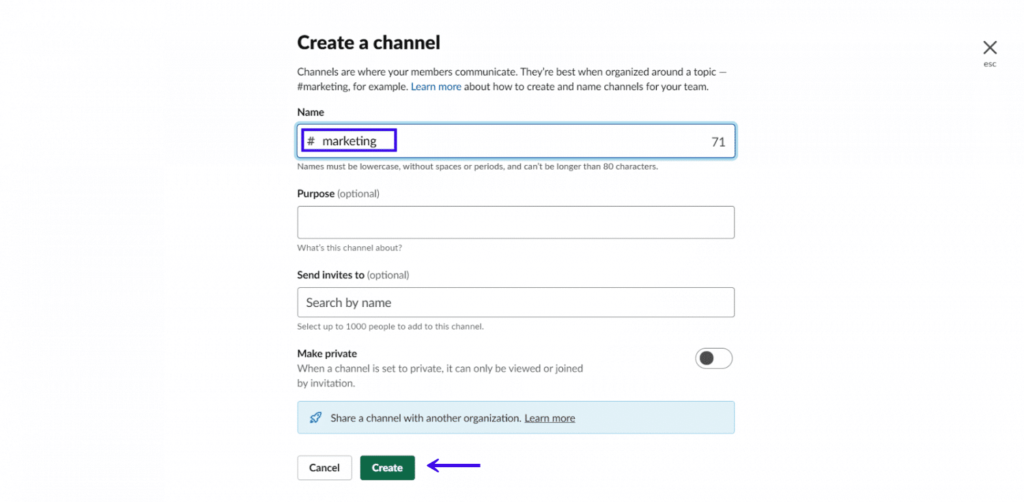On a crisp white background, the page prominently features a user interface for creating a channel. 

In the upper right-hand corner, a gray "X" icon labeled "ESC" indicates an option to close the page. Opposite this, on the upper left, bold black text commands attention with the heading "Create a Channel." Beneath this, slightly less bold gray font informs the user: "Channels are where your members communicate. They're best when organized around a topic, such as #marketing. Learn more about how to create and name channels for your team."

Moving downwards, the user is prompted with a field labeled "Name," which is accompanied by a blue box containing the hashtag "#marketing," distinguished by a purple highlighting rectangle. A note emphasizes, "Names must be lowercase, without spaces or periods, and cannot be longer than 80 characters."

Further down, an optional field titled "Purpose" includes a text box with the placeholder "What's the channel about?" Additional options for sending invitations appear below, with an instruction to "Search by name" in an adjacent search box, and a note stating, "Select up to 1,000 people to add to this channel."

An unselected option to "Make private" follows, explaining that private channels can only be viewed or joined by invitation. Adjacent to this, a blue panel featuring a small blue rocket ship icon encourages users to "Share a channel with another organization" with a link to "Learn more."

At the bottom, two buttons await user action: a white "Cancel" button and a green "Create" button, the latter highlighted by a white text and a purple arrow, drawing attention to the act of channel creation.